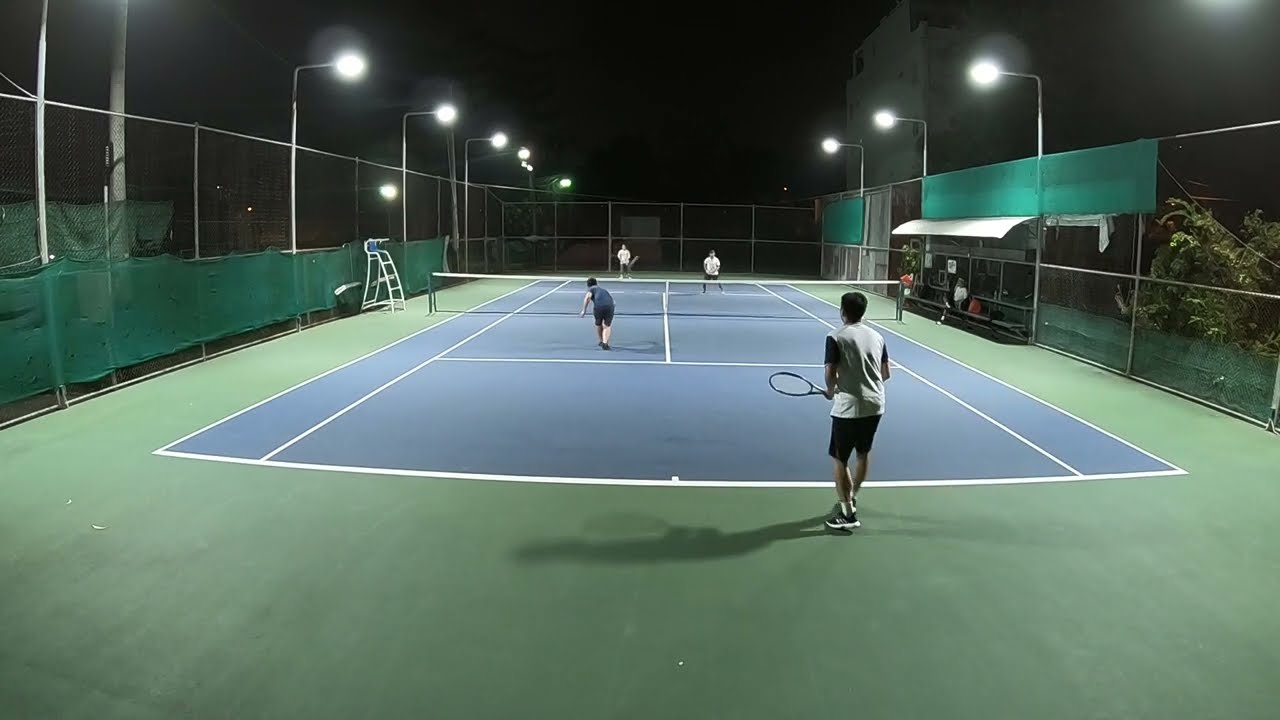In this nighttime scene of an outdoor tennis court, illuminated by multiple circular lights attached to poles, four men are engaged in a doubles match. The court features a blue playing surface bordered by green, with precise white lines marking the boundaries. Surrounding the court is a double chain-link fence, some sections of which have green paneling for added privacy. One team, situated further from the camera, is wearing white shirts. In the foreground, on the right side, a player is dressed in a gray shirt with black shorts, while his partner on the left wears a blue shirt with dark shorts. A shadow can be seen trailing one of the players, indicating recent movement, possibly from a ball being hit. To the right of the court is a bench area under an awning, occupied by onlookers and some bags. One person is seated with their legs crossed, watching the ongoing game. Above, a single star punctuates the black night sky, adding a touch of serene ambiance to the scene. There's also an empty judge's stand prominently visible, hinting at a formal setting. Additionally, trees can be seen in the background, enhancing the outdoor atmosphere.